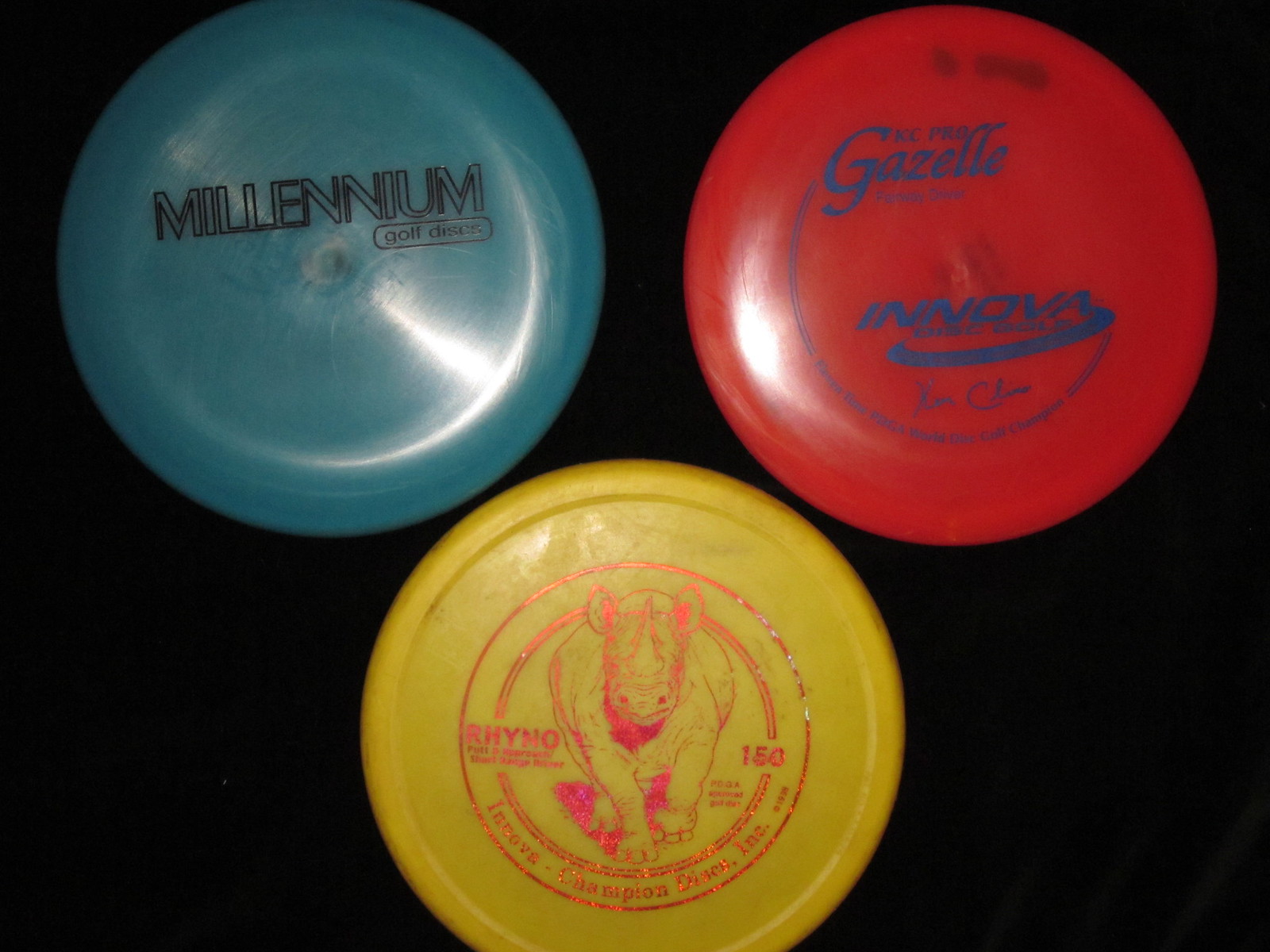This image features three disc golf frisbees arranged against a flat, solid black background, which makes them stand out vividly. The discs are positioned with two at the top and one centered at the bottom. 

- **Top Left Disc:** This is a dark blue plastic disc with the text "Millennium Golf Disc" prominently displayed in black letters.
- **Top Right Disc:** This disc is red in color and bears the text "Gazelle Innova," although the smaller print is difficult to read. It is signed by a person named Ken.
- **Bottom Center Disc:** This is a yellow disc featuring a red print of a rhinoceros with the label "Rhino 150" and the text "Innova Champion" with parts that are hard to decipher.

These frisbees, commonly used in the sport of disc golf, are shown from an aerial perspective and are distinctly shorter than traditional frisbees. This detailed arrangement and presentation highlight each disc's unique color and design elements effectively against the contrasting background.